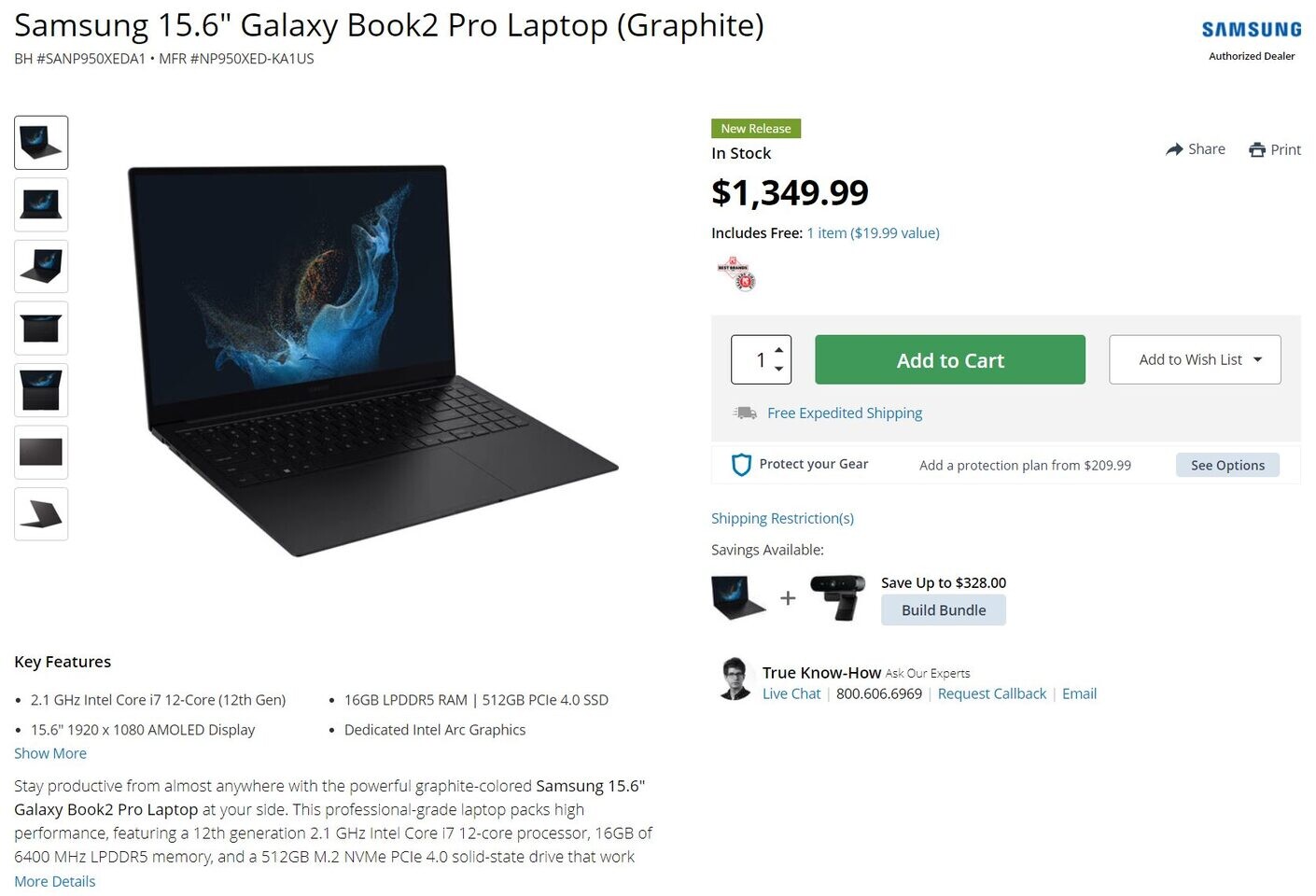This image showcases a sleek Samsung 15.6-inch Galaxy Book 2 Pro laptop in a Graphite finish. The device features a sophisticated, predominantly black aesthetic with a matching keyboard. The laptop's screen is on, displaying a dynamic swirl of blue and yellow hues in the background. Along the left side of the page, a vertical row of thumbnail images offers various viewing angles of the laptop. Beneath the main image, a section titled "Key Features" lists detailed specifications and dimensions. Below this, options to view "More Details" and "Show More" are highlighted in blue, indicating clickable links. At the top, the banner reads "New Release," with the availability status marked as "In Stock." The laptop is priced at $1,349.99 and includes an additional free item. A green "Add to Cart" button and an option to add the product to a wishlist are also prominently displayed.